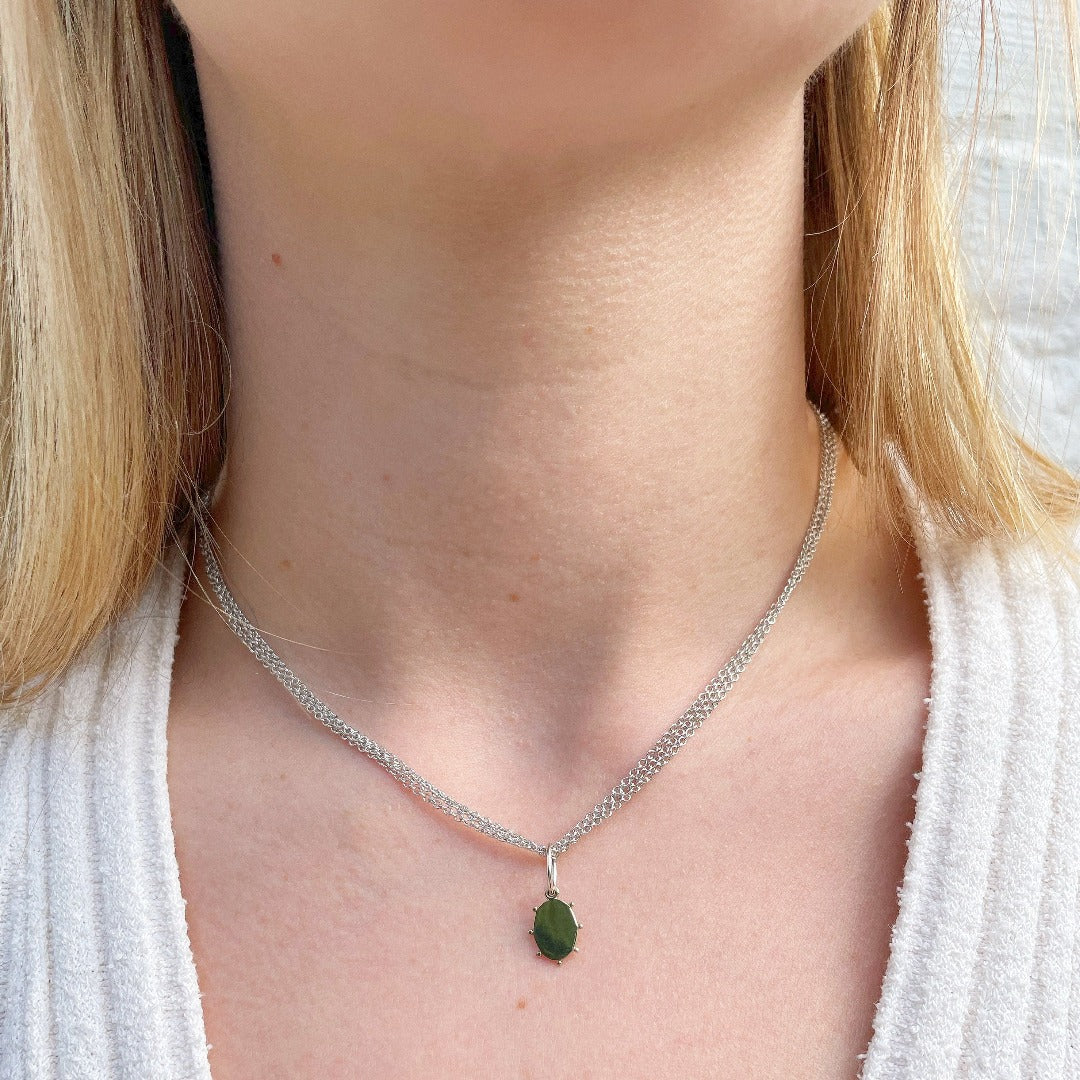This is an up-close photograph of a fair-skinned woman displaying a necklace. You can see her neck, part of her upper chest, and just below her chin. She has shoulder-length, straight blonde hair framing her neckline. She wears a white, v-neck top that resembles a terrycloth robe. The focal point of the image is a delicate silver chain necklace with a small oval pendant. The pendant features a dark green, marbled stone, roughly the size of a fingernail, secured with eight tiny prongs, giving it an appearance reminiscent of a turtle or insect. The background is predominantly white, providing no contextual clues to the setting, and there are a few subtle freckles on her skin, including one just below the pendant and a couple on her neck. This detailed image, possibly from a catalog, emphasizes the elegant necklace.